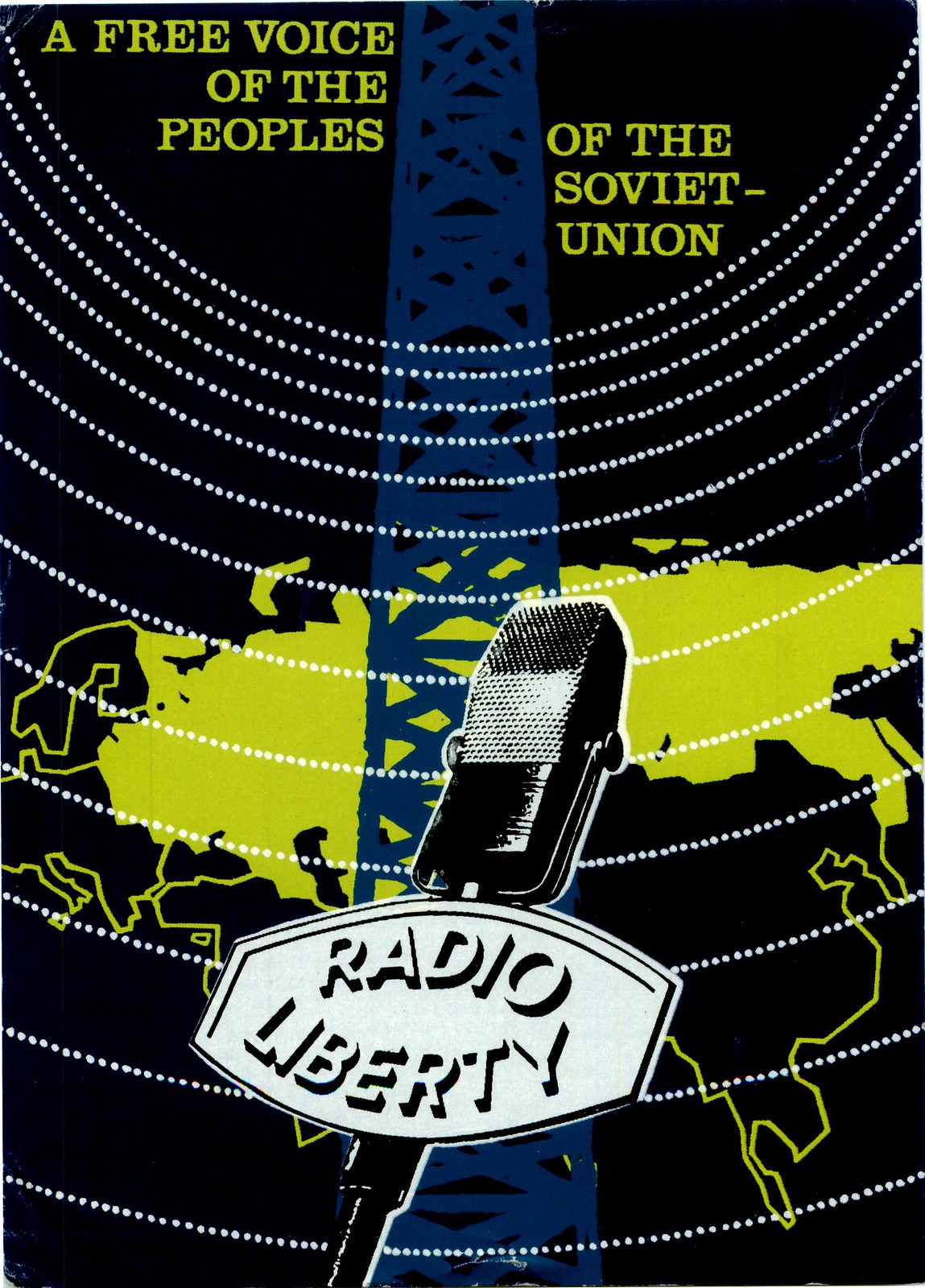The image is a stylized advertisement, resembling a zine or independent magazine cover, with a primarily black background. Central to the composition is a detailed map outline of the Soviet Union, highlighted in a vivid yellow color, set against the larger backdrop of Europe and Asia. Prominently featured in the middle of the image is a dark blue radio tower, extending vertically. This tower is adorned with concentric, ripple-like dotted circles emanating from it, symbolizing radio waves.

At the top left side of the tower, in the same lime-yellow hue as the map, is the text "A Free Voice of the Peoples of the Soviet Union." The phrase continues on the right side, maintaining the lime-yellow color continuity. At the base of the tower sits an old-school black microphone, centrally positioned, with the label “Radio Liberty” displayed in a mix of white and yellow text. The overall aesthetic of the image effectively highlights the Soviet Union and emphasizes the theme of broadcasting freedom through Radio Liberty.